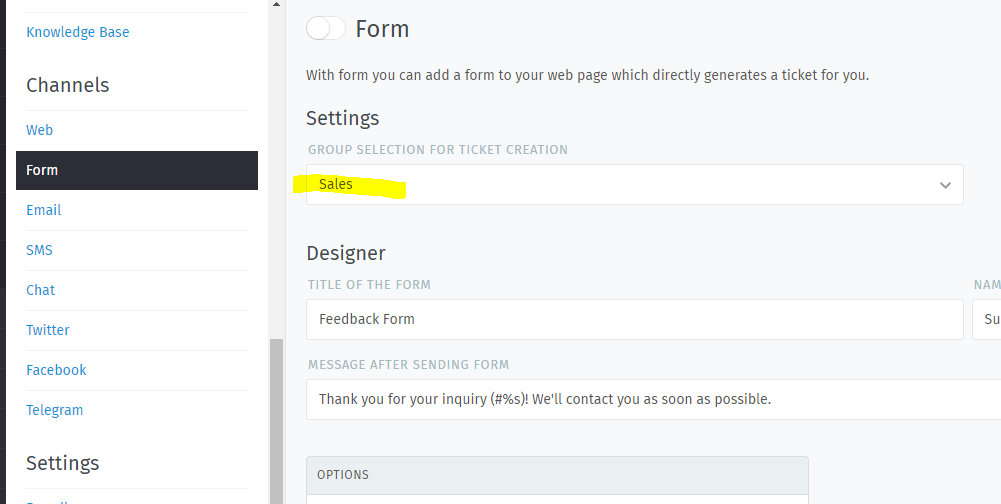The image captures a segment of a web page, likely from the upper right-hand corner, though it does not include the header or topmost section, thus obscuring the name of the company or software. The layout features a dual-color scheme with a primarily white background on the left side, which includes a sidebar menu. The visible portion of the sidebar suggests it is not displayed from the very top. At the top left of the sidebar, "Knowledge Base" is written in blue font. Directly underneath, "Channels" is labeled in black font, followed by a list of items, mostly in blue font except for "Form," which is highlighted in white font against a black background, indicating it is the selected item. Other items listed include "Web," "Email," "SMS," "Chat," "Twitter," "Facebook," and "Telegram," with "Settings" at the bottom in black font.

Occupying approximately three-quarters of the page, the main content area is dedicated to the "Form" interface. The background here is a very light bluish-gray. At the top left, "Form" is labeled in gray font, accompanied by an unselected slider button beside it. Beneath this, a descriptive text reads: "With Form you can add a form to your web page, which directly generates a ticket for you." The next section is labeled "Settings," under which "Group selection for ticket creation" is prominently displayed with a drop-down menu showing "Sales" as the selected option. "Sales" appears to be highlighted with a digital yellow highlighter. Below this is the "Designer" section, followed by the "Title of the Form," with "Feedback Form" entered in the provided box. The section "Message after sending form" features the text "Thank you for your inquiry, we'll contact you as soon as possible" as the selected message. At the bottom, there is a gray rectangle labeled "Options" in gray font.

Finally, a URL "http://TheBusinessProfessor.com" is noted, which may be relevant to the web page in question.